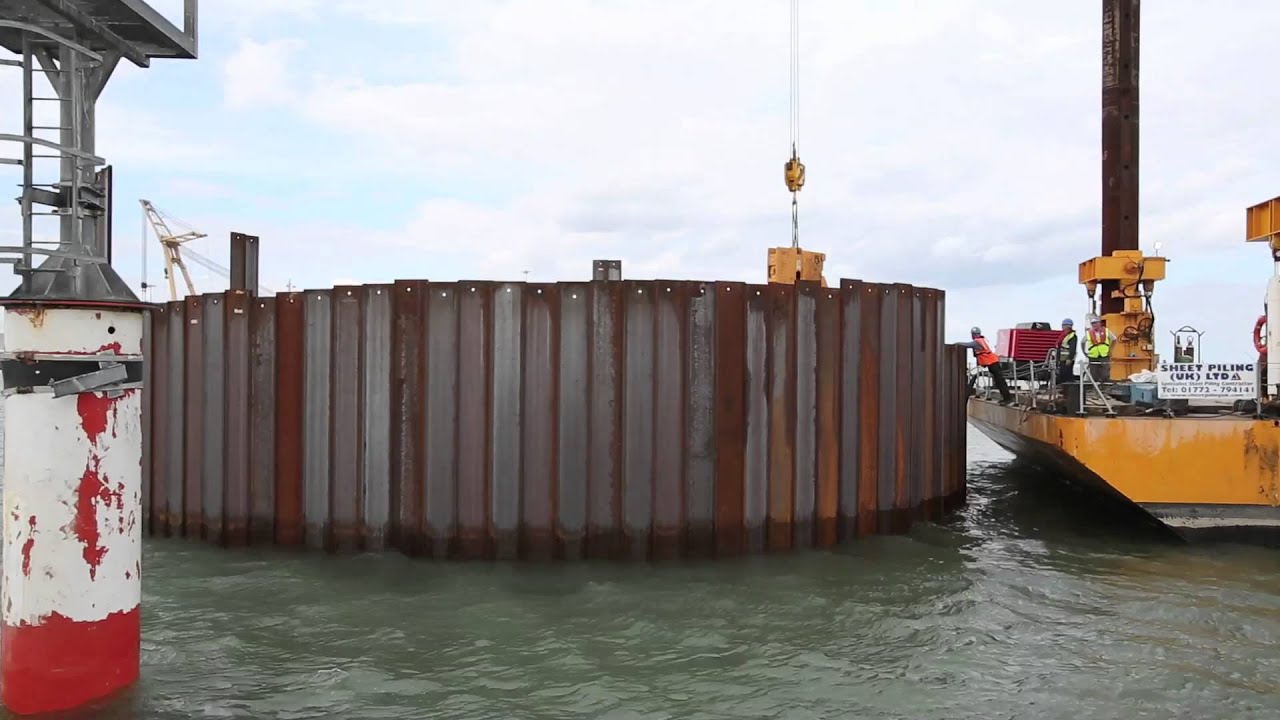This color photograph captures a detailed scene of a maritime construction project. At the center of the image is a circular metal structure, known as a cofferdam, surrounded by green-hued water. The cofferdam comprises numerous steel uprights with small holes at their tops. To the left of the cofferdam, a wall adorned with white paint and patches of red, peeling paint extends down into the water, supported by a metal superstructure. A crane's wires descend over the cofferdam, partially obscuring a yellow object. On the right side of the frame, a yellow barge can be seen, bearing a white sign with the text "Sheet Piling Limited." Several construction workers, clad in high-visibility vests, are standing on the barge, with one laborer leaning on the cofferdam. The backdrop features a cloudy sky, completing this industrial waterfront scene.